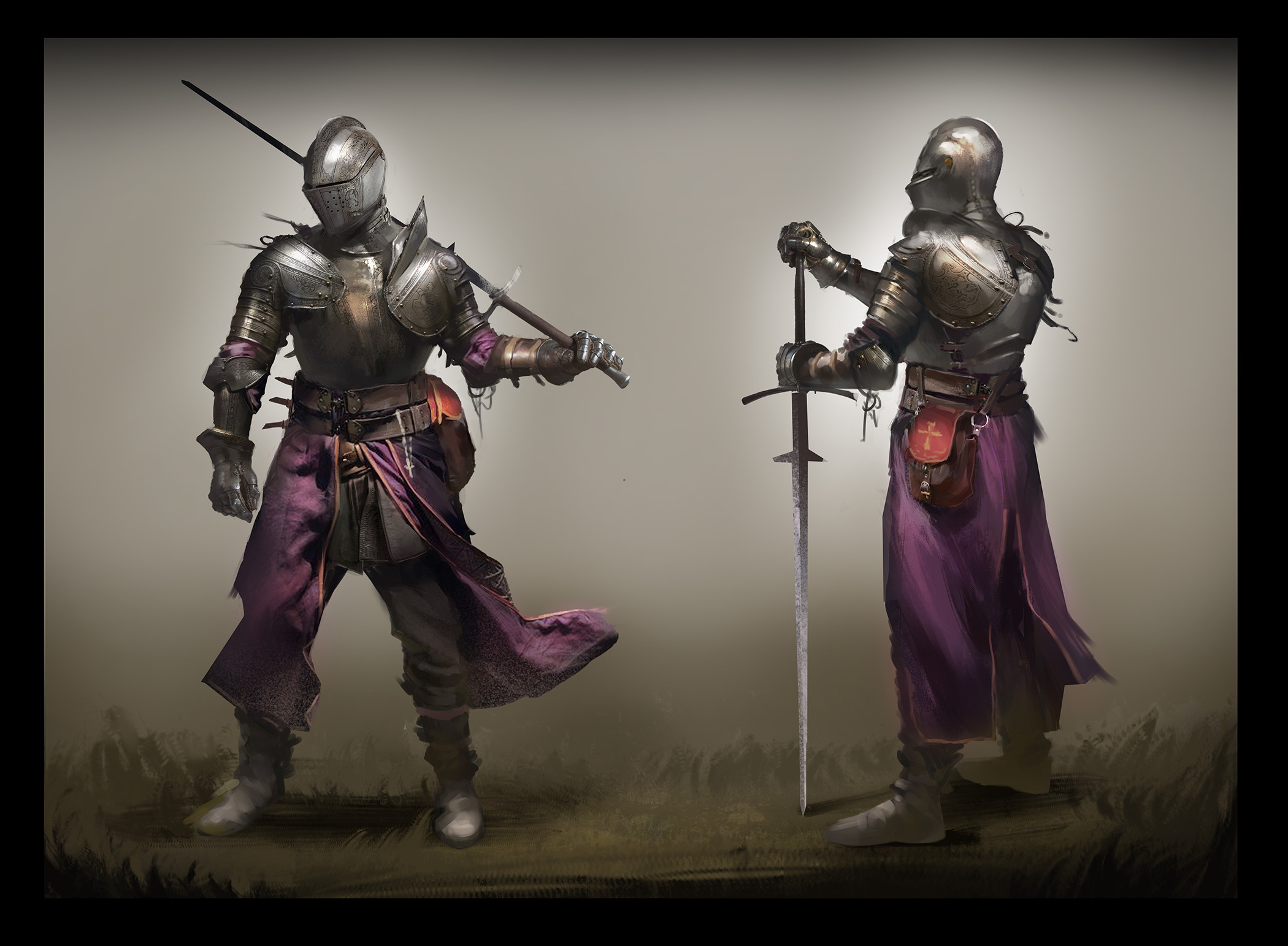The digital drawing presents a front and rear view of a knight dressed in highly polished silver medieval plate armor. The knight, whose face is obscured, wears a vivid purple robe or tunic visible at the elbows and flaring out beneath the double belts at the waist. The rectangular artwork features a thin black border framing the main image, accentuating the gray background and the grass at the bottom, which appears muted and grayish. In both views, the knight grasps a long silver sword. The front view shows the knight facing forward, while the rear view depicts the knight turned away, gazing to the left with the sword pointed downwards. The overall image captures a somber mood with its dark and cloudy sky backdrop, invoking a sense of melancholy in the dull, foggy scene.